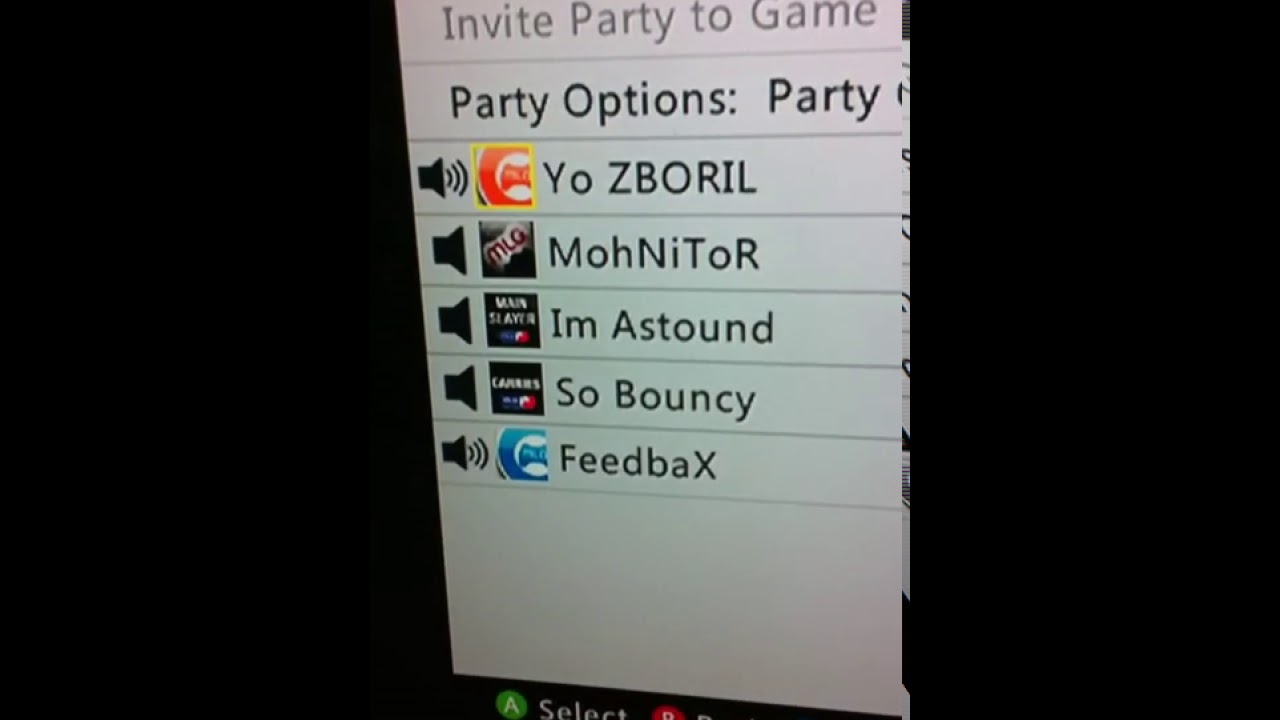The image is a screenshot of a party chat interface from a video game console, likely an Xbox. The screen is predominantly white and centrally aligned with a black background surrounding it. The top of the interface displays "Invite party to game" in gray text, followed by "Party options: Party" in black text. Below these headers are the gamer tags of five users, each accompanied by an audio icon, indicating their voice chat status with some possibly muted and others active. The gamer tags listed are "YO ZBORIL," "MOHNITOR," "IM ASTOUND," "SO BOUNCY," and "FEEDBAX." The bottom of the interface features a green button with an "A" labeled "Select" and a partially visible red "B" button, suggesting options to navigate or start/back functions. The detailed representation suggests a structured and user-friendly UI layout common to Xbox consoles.